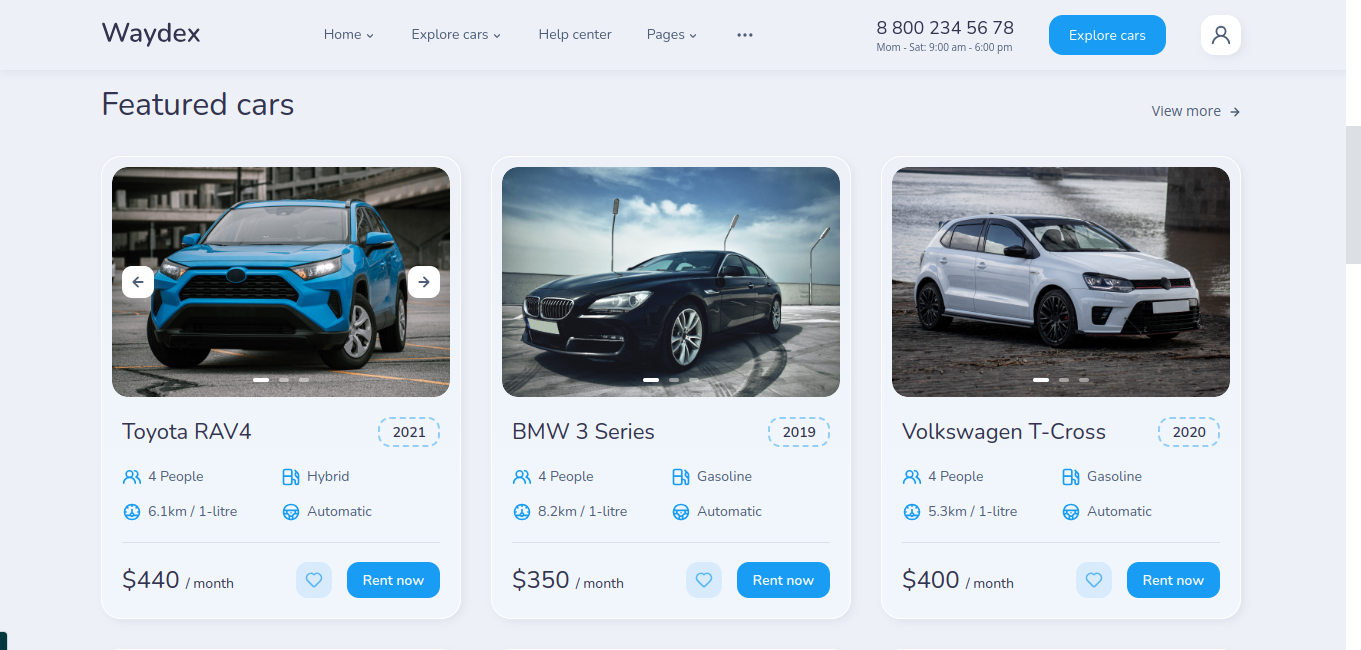This is a detailed descriptive caption for the provided image:

---

The screenshot showcases a website dedicated to cars with a light grey header at the top. On the far left side of the header, the website's logo, "Waydex," is prominently displayed in bold black text. Moving to the right, there are navigation options, each accompanied by a downwards arrow to indicate a dropdown menu. These options, displayed as grey text to the left of the arrows, are labeled as follows: Home, Explore Cars, Help Center, Pages, and a horizontal three-dot menu for additional settings. Adjacent to these, the contact number 8-800-234-5678 is provided, followed by the operating hours, Monday through Saturday, 9am to 6pm. Further to the right, there is a blue "Explore Cars" button with white text, and a white profile picture icon to the far right of the header. A light grey shadow creates a visual separation between the header and the rest of the page.

The body of the page shares a similar grey background color to the header. In the top left corner, the section is labeled "Featured Cars" in bold text. On the top right is a small text link, "View More," with a rightward pointing arrow for additional vehicle listings. Below these headings, three car listings are presented in pop-up cards, each with a high-resolution image and accompanying details.

The first card on the left features a blue Toyota RAV4 parked in an empty parking lot with its wheels turned slightly to the left. Directly below the car's image, it is labeled "Toyota RAV4" with the model year "2021" encased within a blue dashed outline. The card further includes four lines of detailed information, each prefixed by a blue icon: a people icon with the text "4 people," a speedometer icon denoting "6.1 km/1L," a gas pump icon signifying "Hybrid," and a steering wheel icon indicating "Automatic."

---